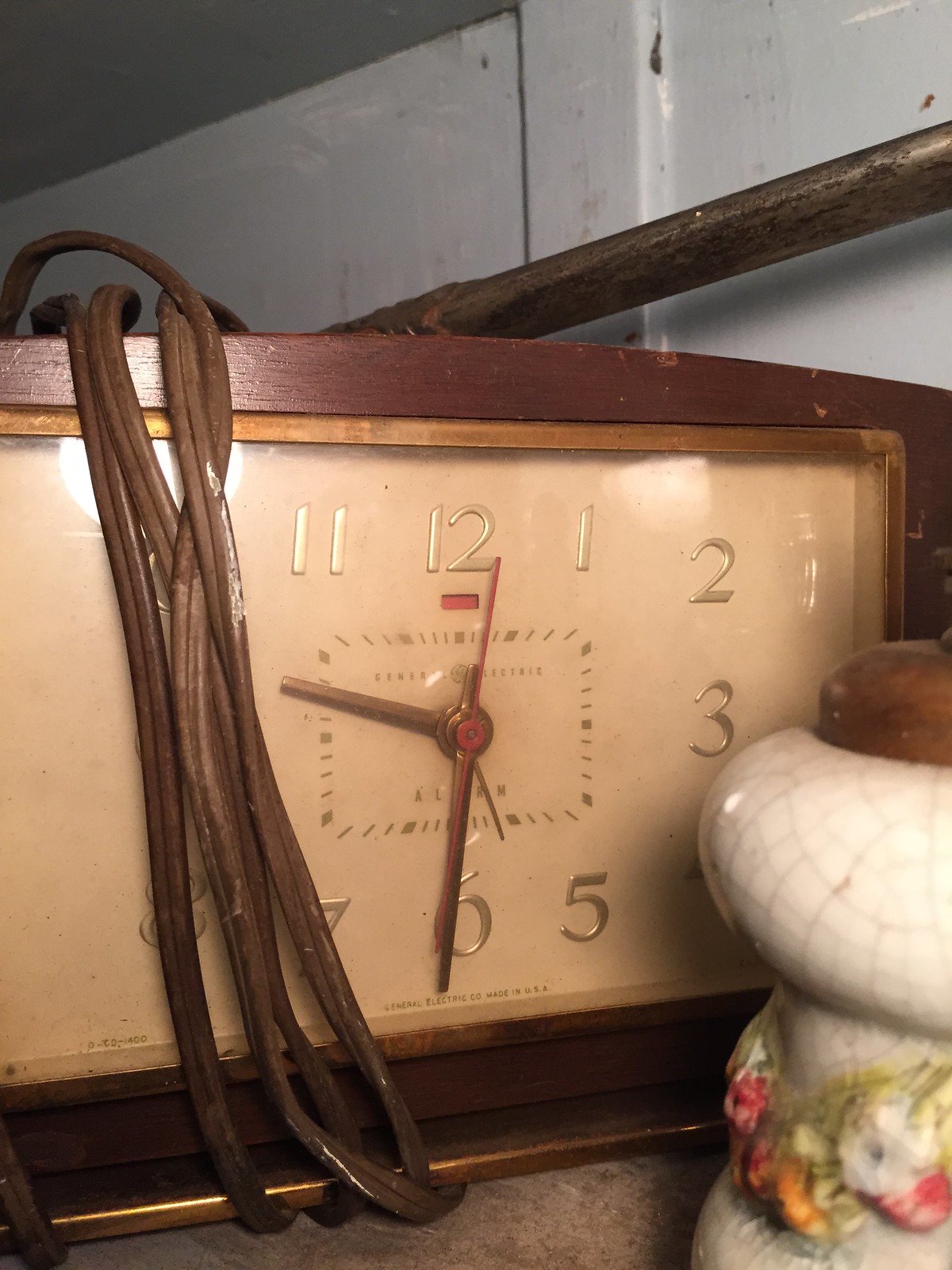A detailed caption for the image:

The image features a rectangular clock prominently centered within a rich, brown wooden frame that transitions to a lighter brown edging. The clock face is rectangular with a beige background. Bronze clock hands mark the time, and golden numbers embellish the face, displaying 11, 12, 1, 2, 3, 5, 6, and 7. Part of the number 8 is obscured by a brown electrical cord, which is wound around the left-hand side of the clock face. To the right-hand corner in front of the clock sits a white ceramic container with visible cracks and a brown top. The container is further adorned with a floral design near its base. Both items rest on a brown table, creating a vintage aesthetic.